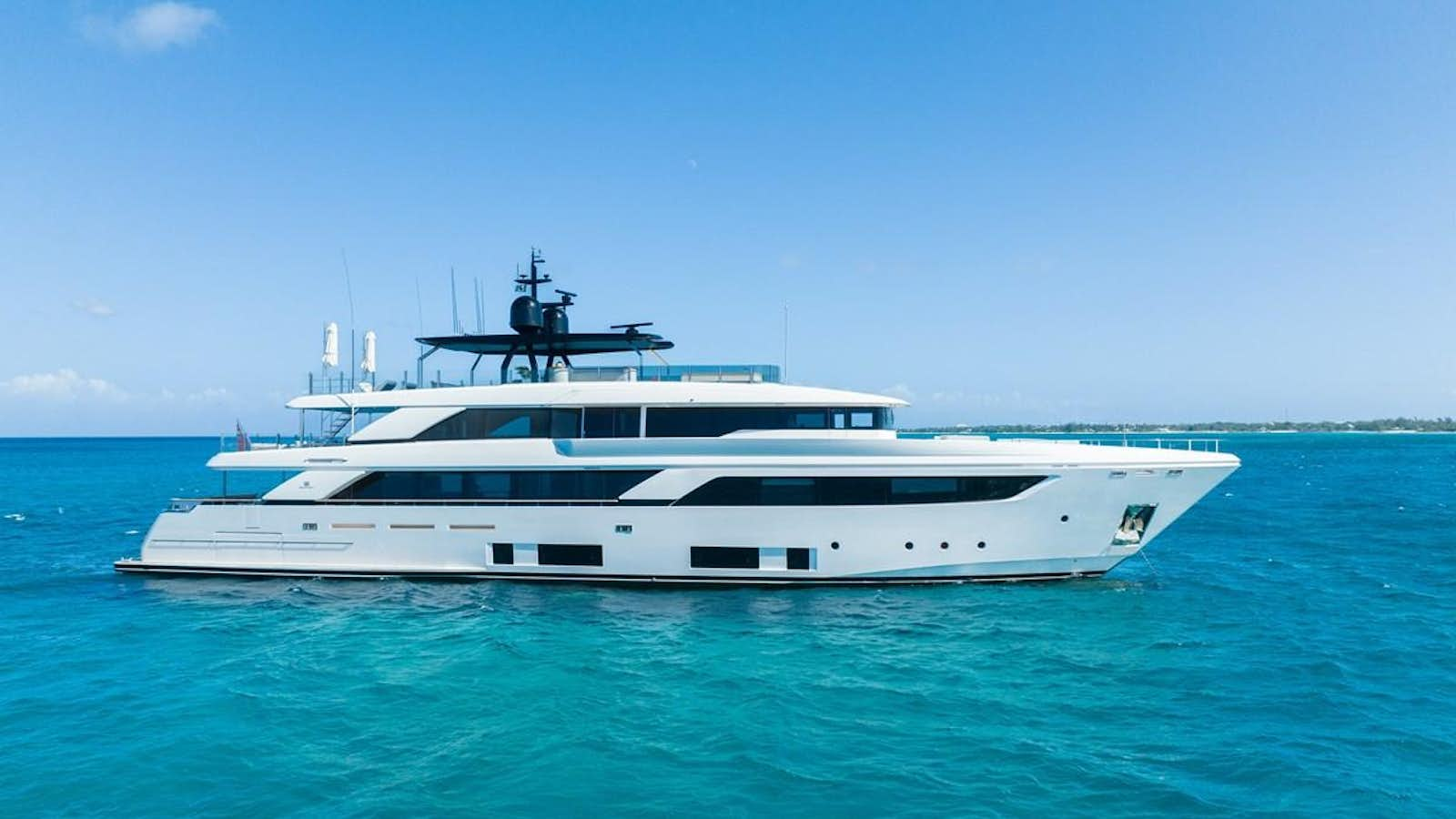This photograph captures a yacht sailing in open, blue waters, possibly in a tropical location like the Caribbean or near Florida or the Bahamas. The yacht, predominantly white with dark windows, is pointing towards the right side of the image. The vessel features three levels, including a deck below. The top deck is distinguished by a flat, black structure with two round elements and a cross-like antenna on top. There are large, rectangular windows spanning across the upper and lower floors, while smaller rectangular windows are visible on the lower deck. In the background, the horizon stretches to the left with a faint tree line visible to the right, suggesting a distant island. The sky above is mostly clear with a few scattered clouds, and a subtle haze adds to the serene atmosphere. A small, indistinct dot appears in the sky, potentially an image artifact or a minor detail.